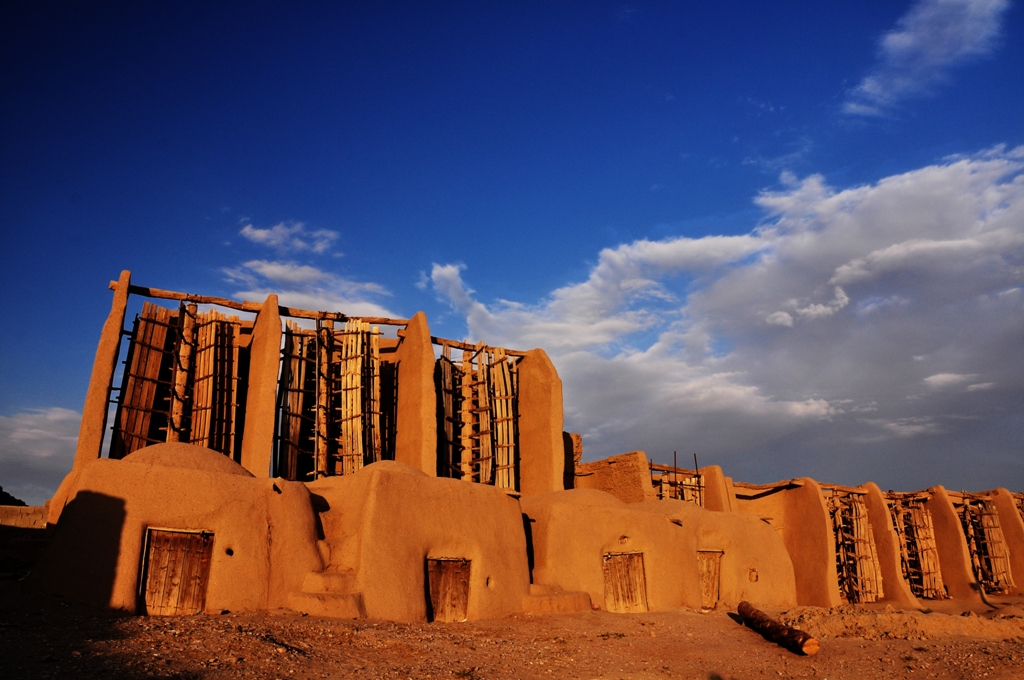An evocative image captures the essence of the Southwest showcasing a series of earth-colored dwellings with distinctive architectural features. These adobe structures have rounded tops with front facades that are more squared off, reflecting traditional design elements. To the right of the buildings, there is an intriguing structure composed of what appears to be bundles of bamboo strung together. This bamboo-like installation is not only adjacent to the dwellings but also extends behind them, arranged in a circular pattern reminiscent of a spin rack’s configuration. While their exact purpose remains unclear, they might serve as elements for energy conservation or wind management. The backdrop features a striking display of fluffy white clouds against a vibrant blue sky, adding a sense of expansiveness to the scene. Complementing these natural and architectural elements, the ground in front of the dwellings consists of earth-toned dirt, punctuated by a single prominent twig in the center bottom of the photograph.